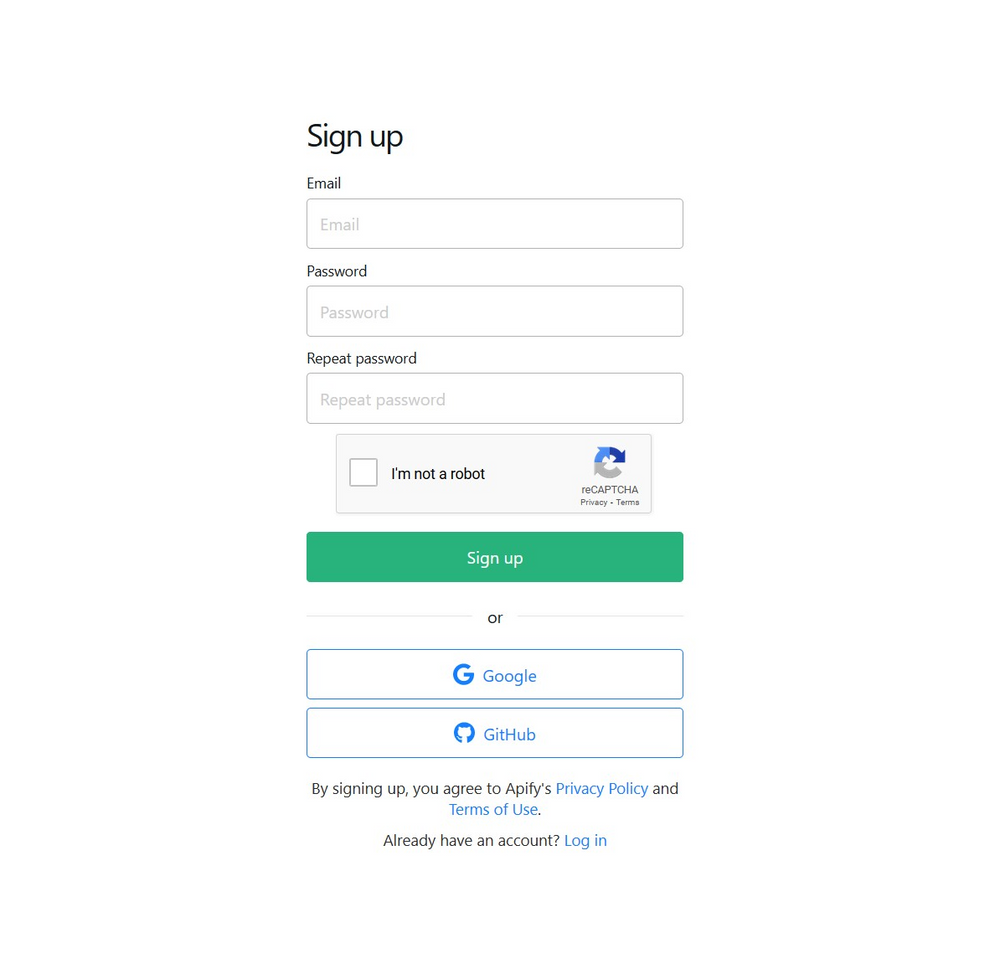In this image, we see a screenshot of a login page on a website, presented in a clean, minimalist design dominated by white space. The interface aims to guide the user through the sign-up process with clear and concise elements. 

At the top left, we are greeted with the prominent text "Sign Up" in bold black letters, indicating the primary action on this page. Directly beneath this, there is a field for entering an email address. This field is a white rectangle bordered by a subtle gray line, and inside it, the placeholder text "Email" is written in gray.

Following the email field, there’s a similar set of text and fields for entering a password. The label "Password" sits above a second white rectangle bordered in gray, with the placeholder text "Password" inside. Moving further down, the interface asks the user to "Repeat Password," which is also above a matching white rectangle with gray text stating "Repeat Password."

Below this sequence of input fields, there is a CAPTCHA verification section. A gray box contains a single checkbox along with the text "I am not a robot." Adjacent to this, there’s a CAPTCHA icon that appears as a clockwise-turning arrow, transitioning from gray to blue, suggesting a dynamic element.

Further down, there is a large green button with white text that invites the user to "Sign Up." Right beneath this button, the word "or" suggests alternative methods for signing up. 

Two additional options are available for sign-up through third-party services. The first is a white rectangle with a blue border, blue text that says "Google," and includes the iconic Google "G." Below this, a similar white rectangle with a blue border states "GitHub" in blue letters, accompanied by a small icon indicative of GitHub's logo.

At the bottom of the page, informational text explains the terms and conditions of using the service: "By signing up you agree to Appify's privacy policy and terms of use." For users who already possess an account, the text "Already have an account? Log in" provides a prompt to redirect them accordingly.

The layout is simple yet comprehensive, offering a user-friendly experience for those looking to sign up to the website.